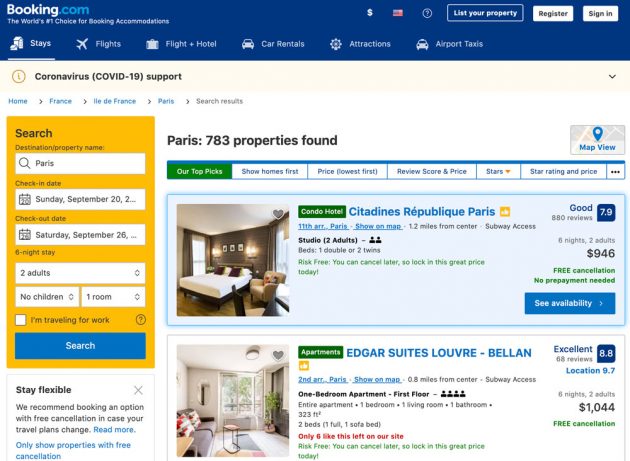Screenshot from Booking.com Interface for Hotel Bookings in Paris: 

The image is a screenshot from the Booking.com website, showcasing the user interface for searching hotel rooms. At the top, there is a distinctive blue navigation bar featuring various icons for booking options such as "Stays," "Flights," "Flight + Hotel," "Car Rentals," "Attractions," and "Airport Taxis." The "Stays" icon is prominently underlined, indicating that the user is specifically searching for accommodation.

In the left sidebar, a yellow rectangle labeled "Search" is visible. Below this, search criteria have been entered: "Paris," with travel dates from Sunday, September 20th to Saturday, September 26th, for two adults with no children. An additional blue "Search" button is located at the bottom of this sidebar.

The main content area displays search results. It is noted at the top of this section that 783 properties have been found in Paris. The user has selected the "Our Top Picks" filter, highlighted in green.

Two specific hotel options are displayed:

1. Condo Hotel - Citadines République Paris: This option is listed at $946 for a six-night stay.
2. Apartments - Edgar Suites Louvre - Bellin: Priced at $1,044 for the same duration of six nights for two adults.

The overall layout and details provide a clear and user-friendly interface for comparing hotel options in Paris.